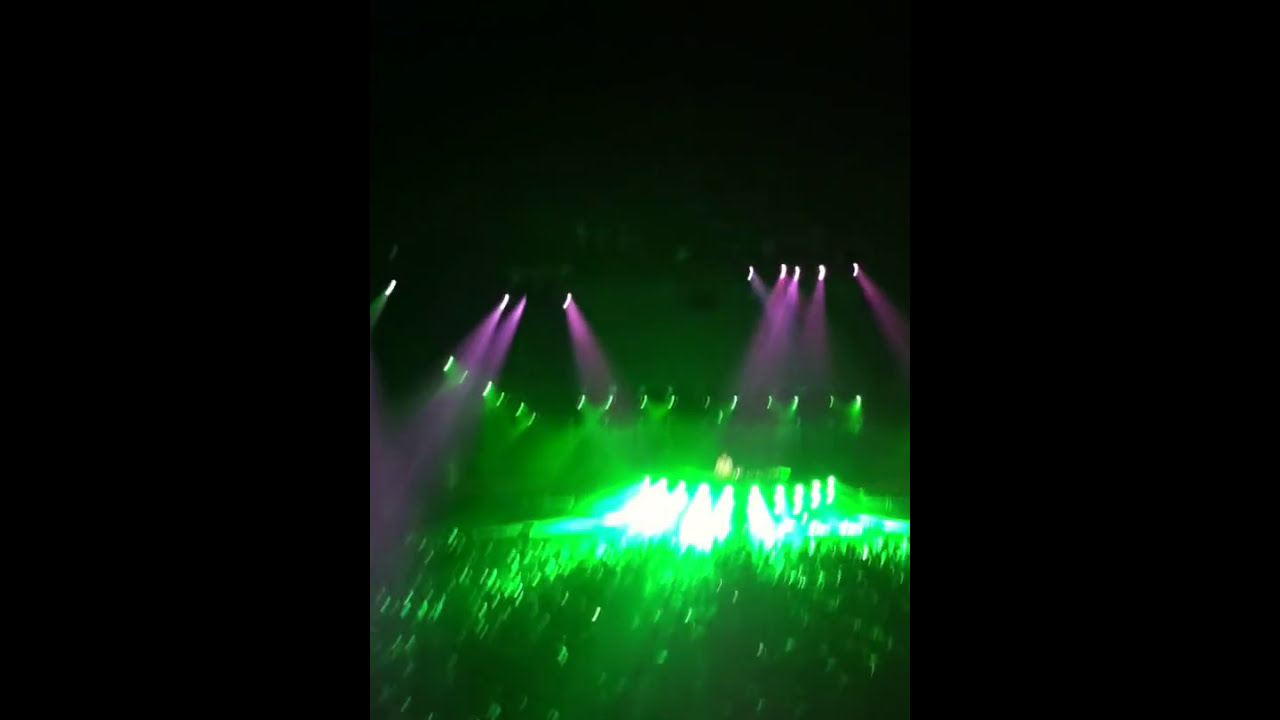The blurry image captures the vibrant, chaotic energy of a concert or show, primarily bathed in green light. At the center of the stage, a blinding concentration of incandescent white and yellow lights dominates, creating an almost ethereal glow amidst the low-quality blur. The top portion of the image is shrouded in darkness, punctuated only by approximately nine spotlights emitting purplish-pink hues in various directions from the ceiling. Additional yellow and orange lights intermingle with the green, particularly at lower positions, casting fragmented reflections over the indistinct silhouettes of the crowd below. There's an impression of a DJ setup on stage, hinted at by a lone figure behind the dazzling lights, reinforcing the show's dynamic and immersive atmosphere.